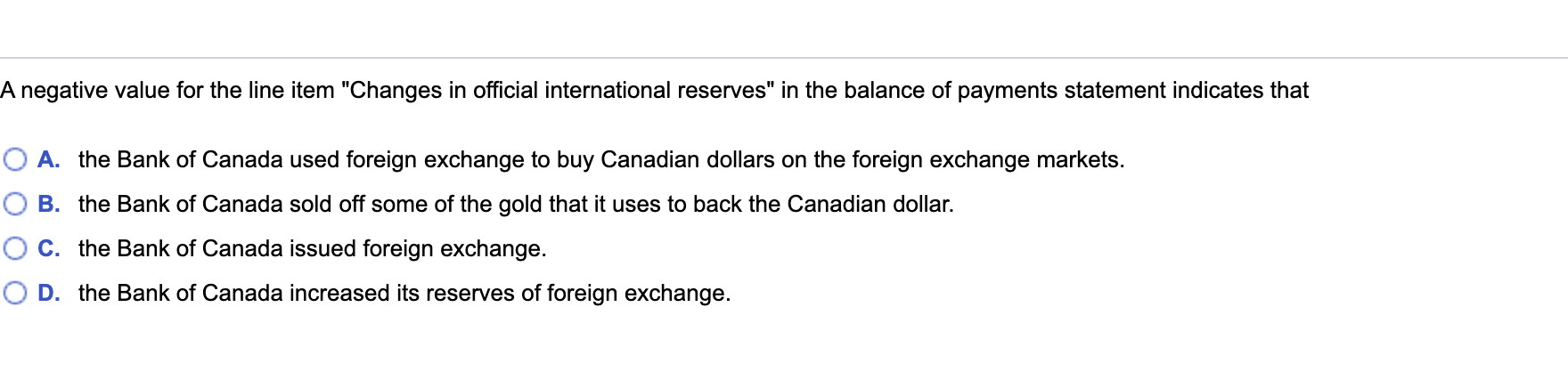The image depicts a section of a multiple-choice test question focusing on macroeconomic policies. At the top of the image, there's a faint gray horizontal line followed by the statement, "A negative value for the line item, 'changes in official international reserves' in the balance of payments statement indicates that:" 

Below this statement, the four answer options are aligned vertically:

- Option A: Highlighted in blue, it includes a blue circle and the letter "A". It states, "The Bank of Canada used foreign exchange to buy Canadian dollars on the foreign exchange markets."
- Option B: Also highlighted in blue with a corresponding blue circle and the letter "B". It states in black text, "The Bank of Canada sold off some of the gold that it uses to back the Canadian dollar."
- Option C: Following the same format, it is highlighted in blue with a blue circle and the letter "C". It states in black text, "The Bank of Canada issued foreign exchange."
- Option D: The final option highlighted in blue, features a blue circle and the letter "D". It states in black text, "The Bank of Canada increased its reserves of foreign exchange."

Each option ends with a period. The answer choices illustrate various actions that can affect the balance of payments by the national bank.